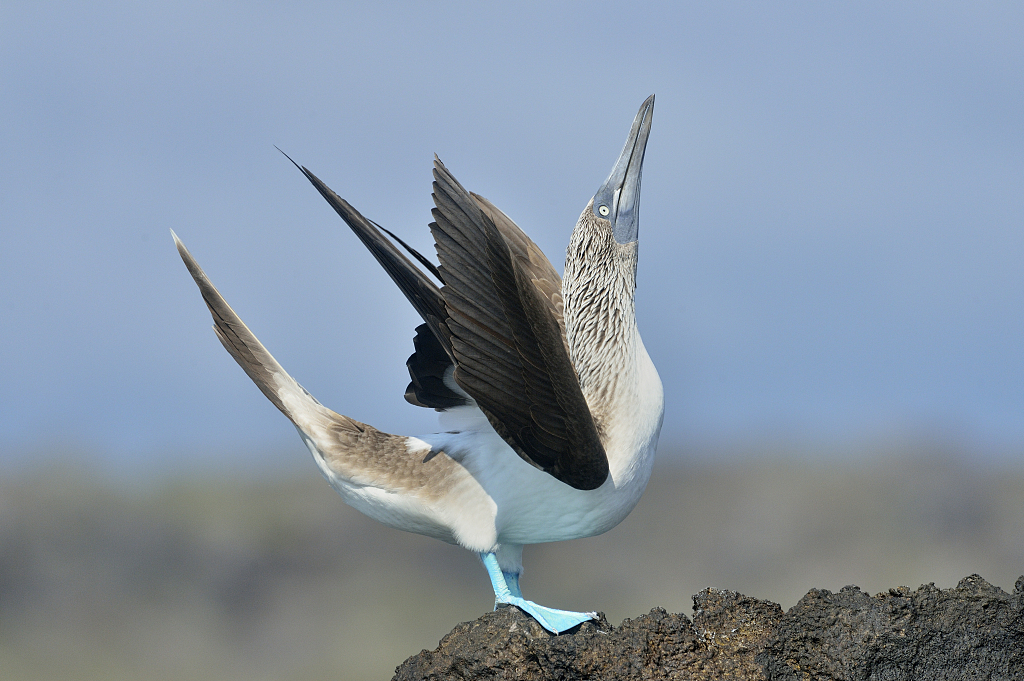The image captures a professional, full-color photograph taken outdoors on a sunny day using natural light. The horizontally rectangular photo is without a border and depicts a striking scene under a blue sky, occupying most of the top portion of the image. The bottom third reveals a ridge of dark brown rocks, particularly concentrated in the lower right corner and spreading towards the middle bottom. Perched on this rocky formation is a distinctive bird engaged in an upright posture, with its long, pointy beak stretched skywards, neck elongated, and wings outstretched. The bird showcases a unique palette: a predominantly gray back and neck, with baby blue or teal tinges along its belly, transitioning to white on its body. It has coarse feathers around the neck, black wings, dark tail feathers, and light blue webbed feet, indicative of its aquatic nature. The blurred background and the detailed foreground highlight the bird's striking features and dynamic pose against the clear sky and rugged terrain.